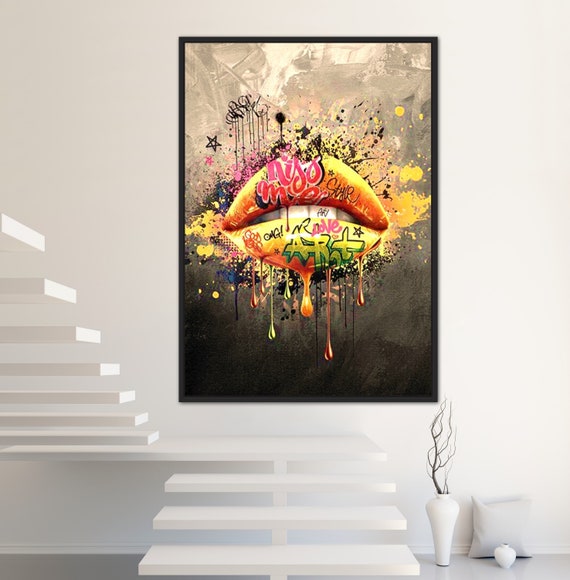The photo captures a stylish and modern interior. The focal point is a striking abstract art piece on a large, white wall. The artwork features a prominent pair of yellow-orange lips, reminiscent of graffiti, with bold pink text saying "KISS ME." The lips also have colorful drips in blue, yellow, green, orange, and red, with additional blotches and spatters of black, blue, yellow, orange, pink, and stars scattered around. The framed art stands out against the minimalist background of white walls.

In front of the wall art is a set of floating, modern white wooden stairs. These stairs take a slight curve as they ascend and appear almost precarious due to their lack of handrails, contributing to a very open and minimalist aesthetic. The stairs look as though they are comprised of pieces of wood stacked together with minimal support.

The lower right of the image shows a small decorative white pillow on the floor, a tiny empty vase, and a larger white vase holding a barren tree branch, likely a curly willow. A trash can is also visible in the lower right corner, adding a subtle touch of everyday reality to the chic setting. The image emphasizes stark contrasts and clean lines, encapsulating a contemporary and avant-garde atmosphere.